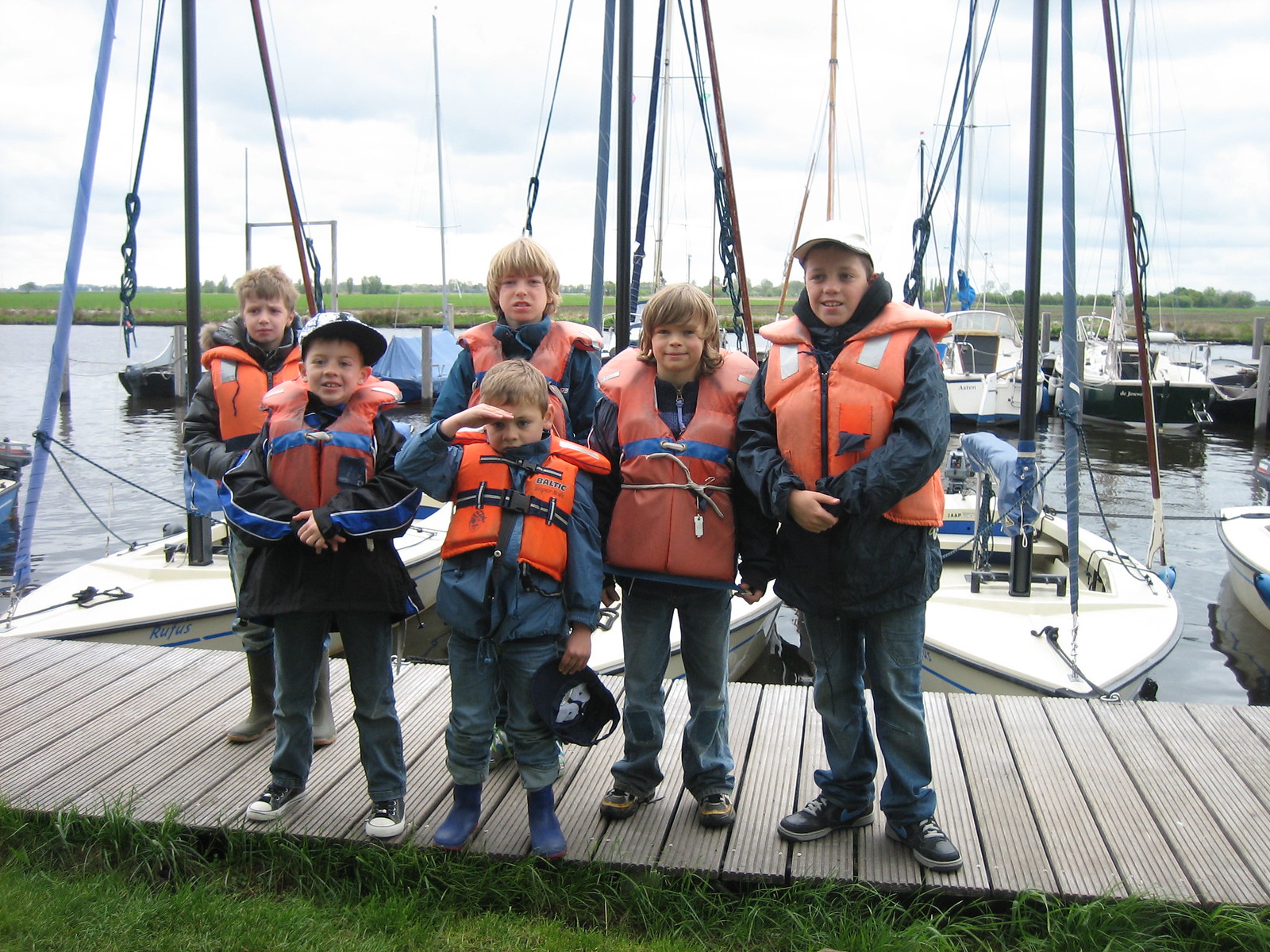A vibrant group photo captures six boys, all under the age of 11, gathered on a wooden dock at a marina, poised and ready for a boating adventure. The dock is characterized by light brown, almost gray wooden panels, each adorned with vertical lines for added grip. The children, clad in bright orange life vests—some more faded and dirtier than others—are bundled up in long-sleeved jackets and jeans, indicating a chilly, overcast day. Their footwear varies from sneakers to boots, emphasizing their preparedness for outdoor activities. Two boys, positioned at the front and back, sport baseball caps, with one of them playfully saluting and holding his cap. Behind them lies a serene scene of medium to small sailboats, moored along the dock and dotting the still waters of the lake, which is bordered by a stretch of green grass and trees in the distance. The sky is shrouded in white clouds, adding to the overall muted, yet lively ambiance of this picturesque moment. All the boys have blonde hair, with most having a shaggy style, and they share fair complexions and a mix of expressions, from cheerful to pensive, suggesting a mix of excitement and curiosity for the day’s upcoming adventures.